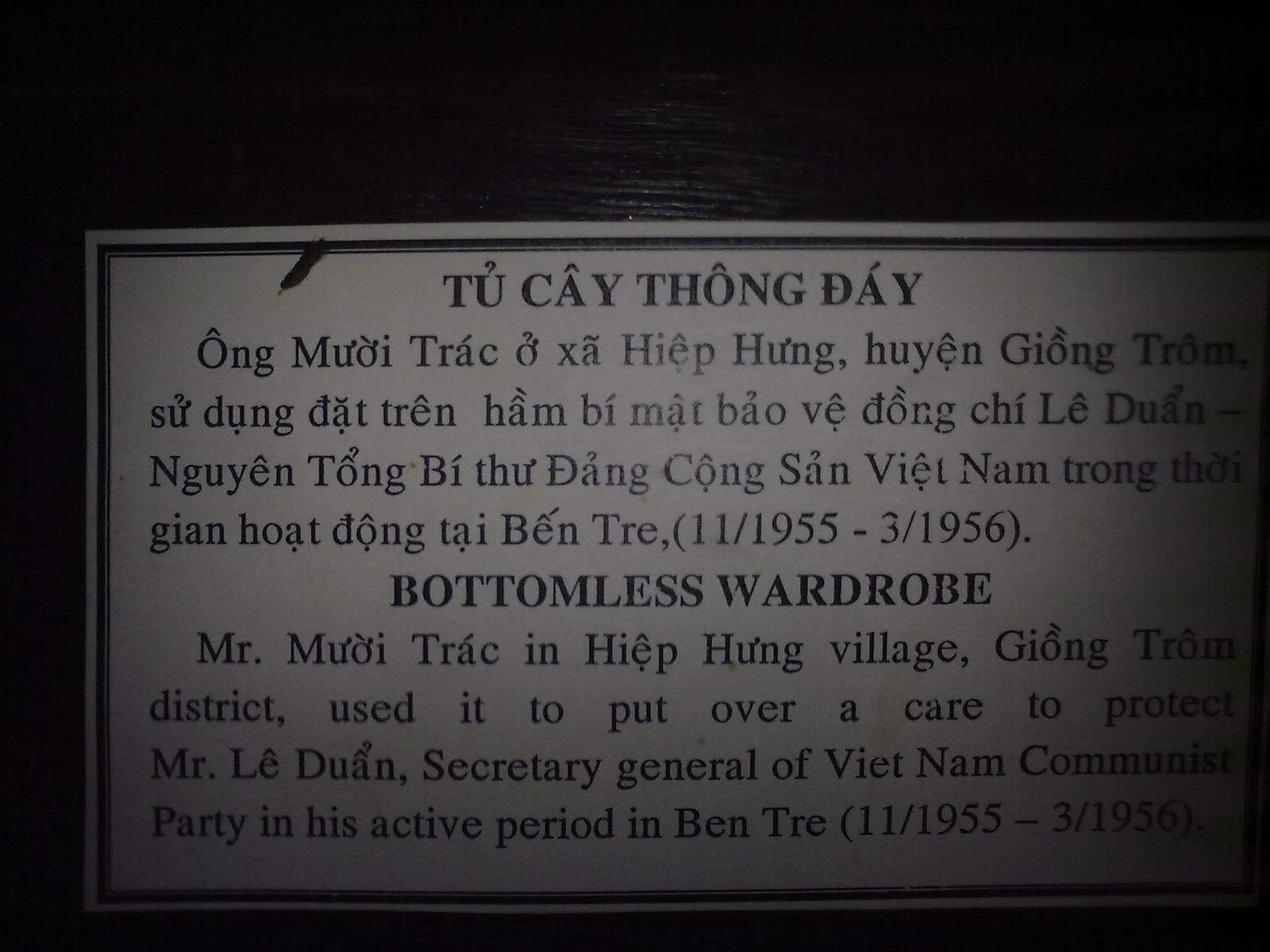The image depicts a commemorative plaque or sign, centrally placed on a dark wood table. The plaque features a piece of paper bordered in black, taking up approximately the bottom three-fourths of the frame, while the top quarter showcases the wood grain of the table. The paper is predominantly white with black text, split into two sections: the upper half is written in Vietnamese, and the lower half provides an English translation. The translated text reads: 

"Bottomless wardrobe. Mr. Mieu Trac in Hiep Hung Village, Duong Troi District used it to protect Mr. Le Duong, Secretary General of the Vietnam Communist Party during his active period, November 1955 to March 1956."

The plaque appears to commemorate an event or individual significant to Vietnamese history, specifically relating to efforts made to ensure the safety of Mr. Le Duong.